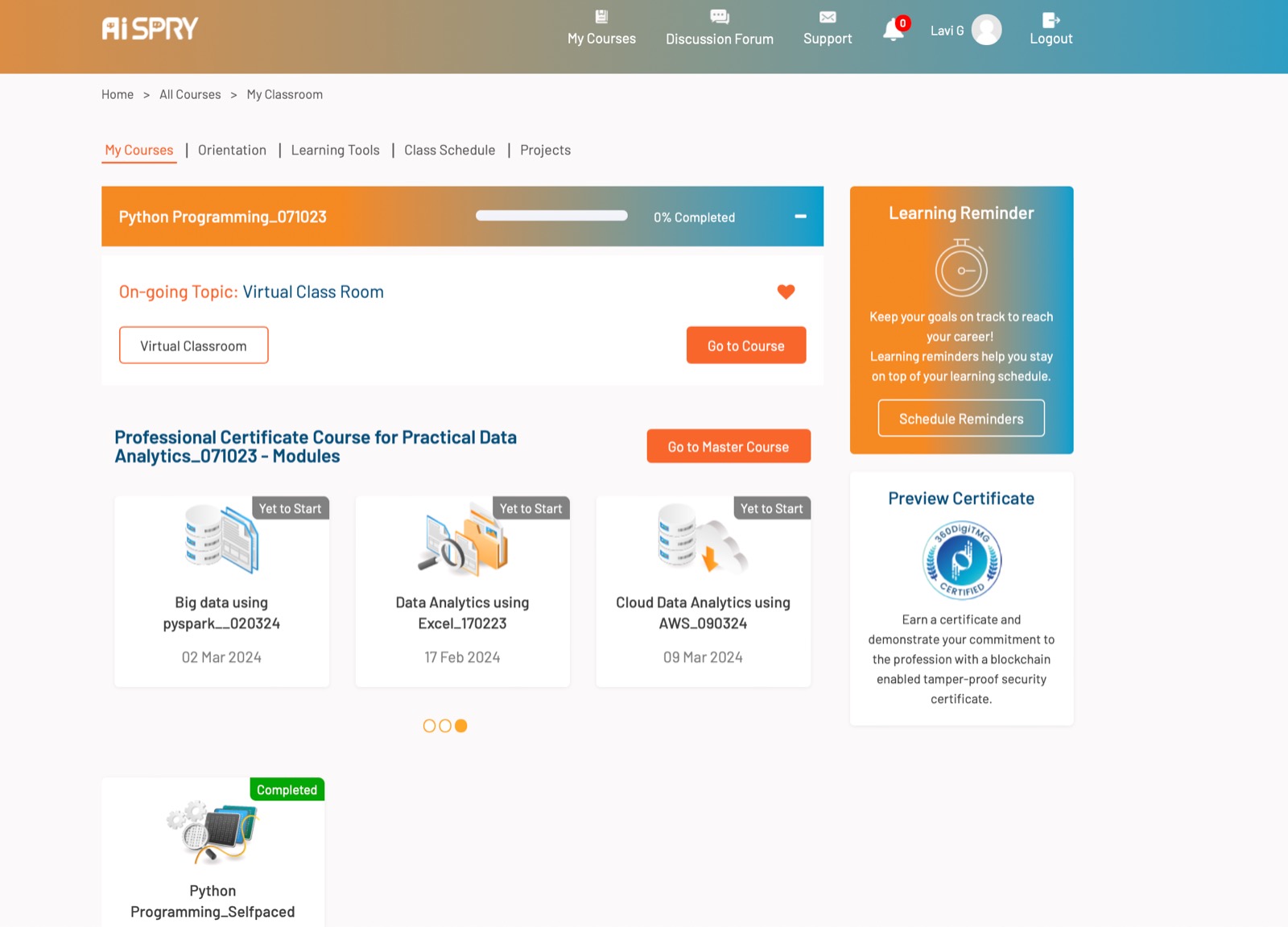This webpage serves as a platform for selling data analysis services and courses. Featured prominently are tabs for various specialized courses: "Big Data Using SciSpark," "Data Analytics Using Excel," "Cloud Data Analytics Using AWS," and a "Python Programming Self-Paced" course, the latter of which appears to be completed. Users can navigate to the coursework through the "Home," "All Courses," and "My Classroom" sections.

The webpage design includes a distinctive top border that transitions from orange on the left to a darker blue on the right. This color gradient is echoed by another bar mid-page and an adjacent image that shares the same color scheme. The text throughout the site displays in diverse colors, including gray, black, blue, and white, creating a vibrant and varied visual experience.

Additionally, there is a "Preview Certificate" link, presumably allowing users to view certificate samples issued upon completing courses. The platform is branded as "AI Spry."